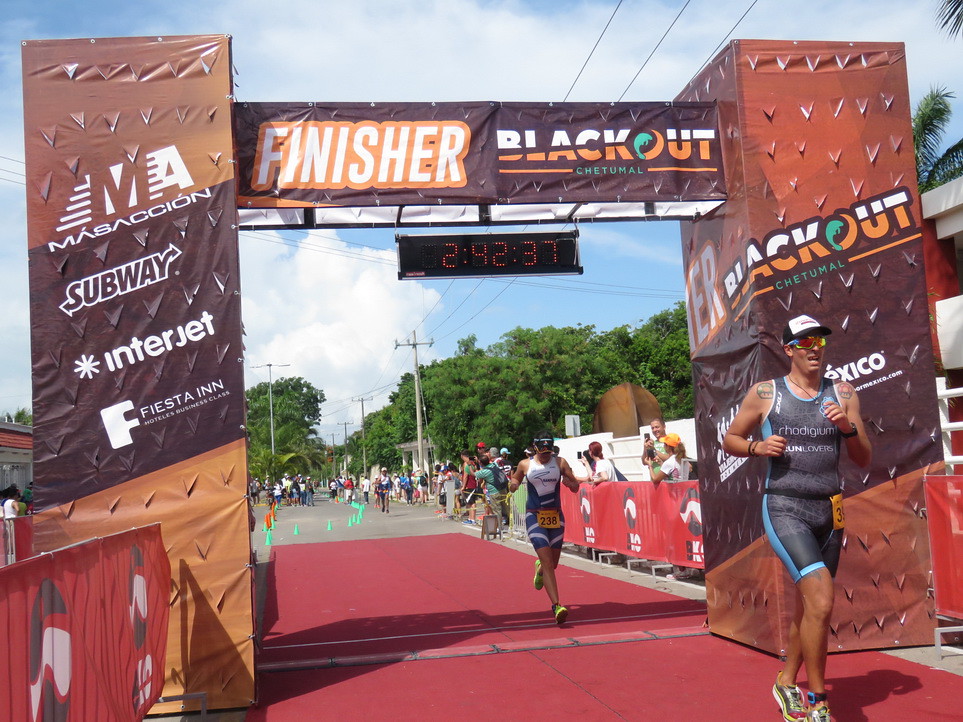The image captures the finish line of a marathon set outdoors on a sunny day with a blue sky dotted with white clouds. Two tall columns rise from the bottom to the top of the image, adorned with advertisements for Interjet, Fiesta N, Subway, and Master Cyan. These columns are connected at the top by a horizontal banner that reads "Finisher Blackout." Below the banner, an electronic clock with orange numbers on a black background displays the time as 2:42:37. A red carpet covers the ground at the finish line area. In the foreground, a male runner wearing a gray tank top, gray shorts, white hat, and sunglasses has just crossed the finish line. Right behind him, another runner in a white and blue tank top and shorts is about to finish. Spectators stand behind a short fence with advertisements, taking photos and cheering the runners. The street continues into the distance, lined with onlookers and bordered by trees and power poles to the right and left.